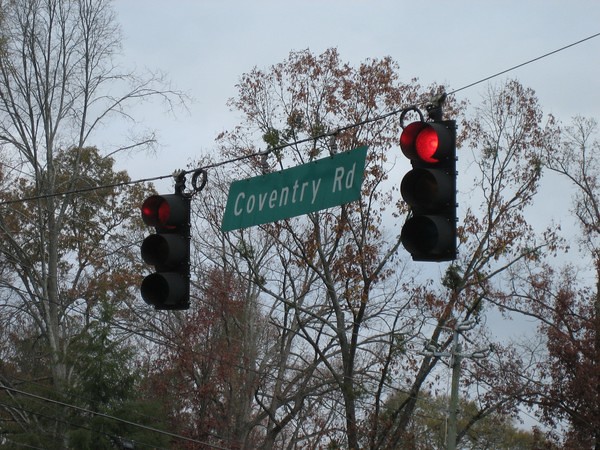The image depicts an older version of a stoplight system, possibly from the 1980s or early 2000s. It features two traffic lights, one on each side, hanging from a relatively thin wire. Each light has the traditional three sections for red, yellow, and green signals, with both lights currently showing red. Suspended between the lights is a green rectangular street sign with white text that reads "Coventry Road, RD." The surroundings hint at winter or early spring, as the trees in the background have a mix of bare branches and some with light green and dark leaves, while one tree displays red leaves or branches. The scene is set against a slightly gray sky, suggesting an overcast day. The overall atmosphere, possibly captured around dusk, lends a softer light to the image, enhancing the sense of an older, serene setting.